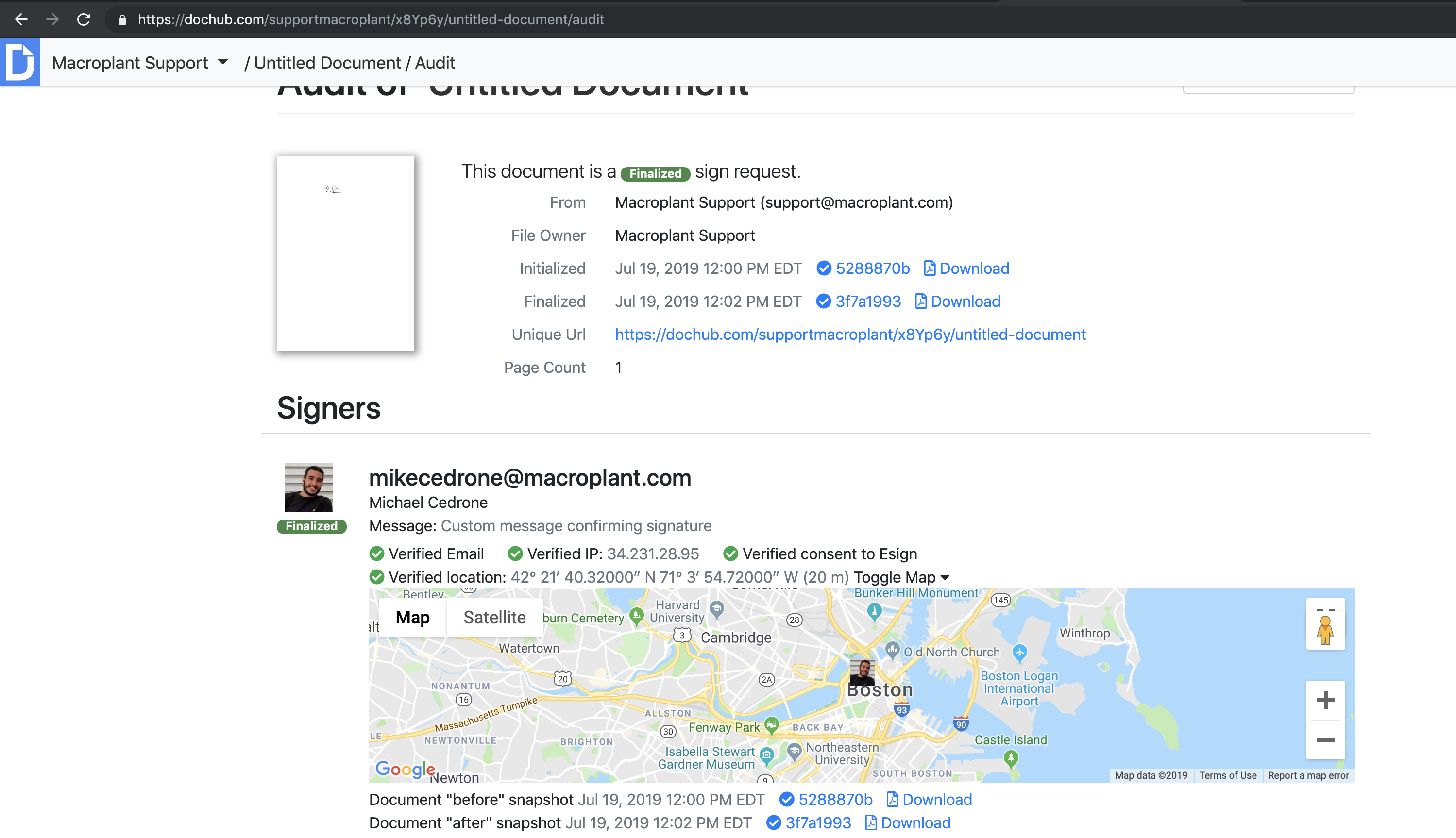This image depicts a web page displaying a finalized, signed request from Macroplan Support. The URL visible in the browser reads: ".gov.com/supportmacroplan.com/XBYP6Y/untitled-document/audit". The header of the page indicates "Macroplan Support" and the document status as "Audit Affirmative".

The document shown is titled "Untitled Document / Audit". It represents an officially signed request from Macroplan Support, with the email address support@macroplan.com listed as the file owner.

Details of the document's timeline are as follows:
- Date of Initialization: July 19th, 2019, at 12:00 PM.
- Date of Finalization: July 19th, 2019, at 12:02 PM.

The document was signed by mikecidrone@macroplan.com. Additionally, the document includes a detailed map of a specific area in Boston.

The process for sending this document for electronic signature (eSign) is documented, with the verified IP address noted as 34.231.28.95. The location verification is also confirmed for added security and authenticity.